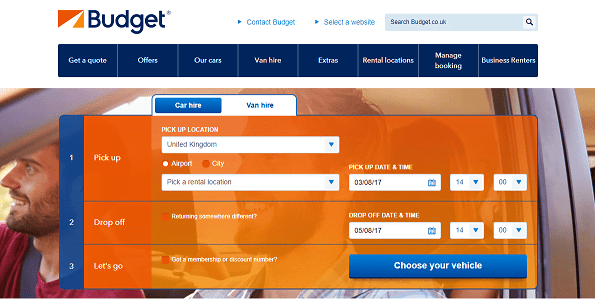This is a detailed description of a screenshot taken from the Budget website. The top-left corner of the interface prominently displays the "Budget" logo, characterized by an orange rectangle intersected by a white triangle. Beside the logo, there are two blue buttons labeled "Contact Budget" and "Select the Website," as well as a search bar reading "searchbudget.co.uk."

Immediately beneath this header, a navigation bar includes tabs for "Get a Quote," "Offers," "Our Cars," "Van Hire," "Extras," "Rental Locations," "Manage Booking," and "Business Renters." Below the navigation bar, there's a vehicle selection interface dominated by various fillable fields. The website employs an orange, royal blue, and navy blue color scheme, with a predominantly white background for contrast.

In the background of this section, there is an image of two men driving a car, both smiling. The central card, which is orange and blue, features two selectable tabs labeled "Car Hire" and "Van Hire," with "Car Hire" currently active. The card outlines a three-step process for booking: "Pickup," "Drop Off," and a final step labeled "Let's Go."

For the "Pickup" step, users are prompted to fill in the pickup location, date, and time, with additional fields for related information. The "Drop Off" step requests the drop-off date and time, accompanied by further details indicated by additional checkmarks. Beneath these steps, a blue button labeled "Choose Your Vehicle" invites users to proceed with selecting a vehicle.